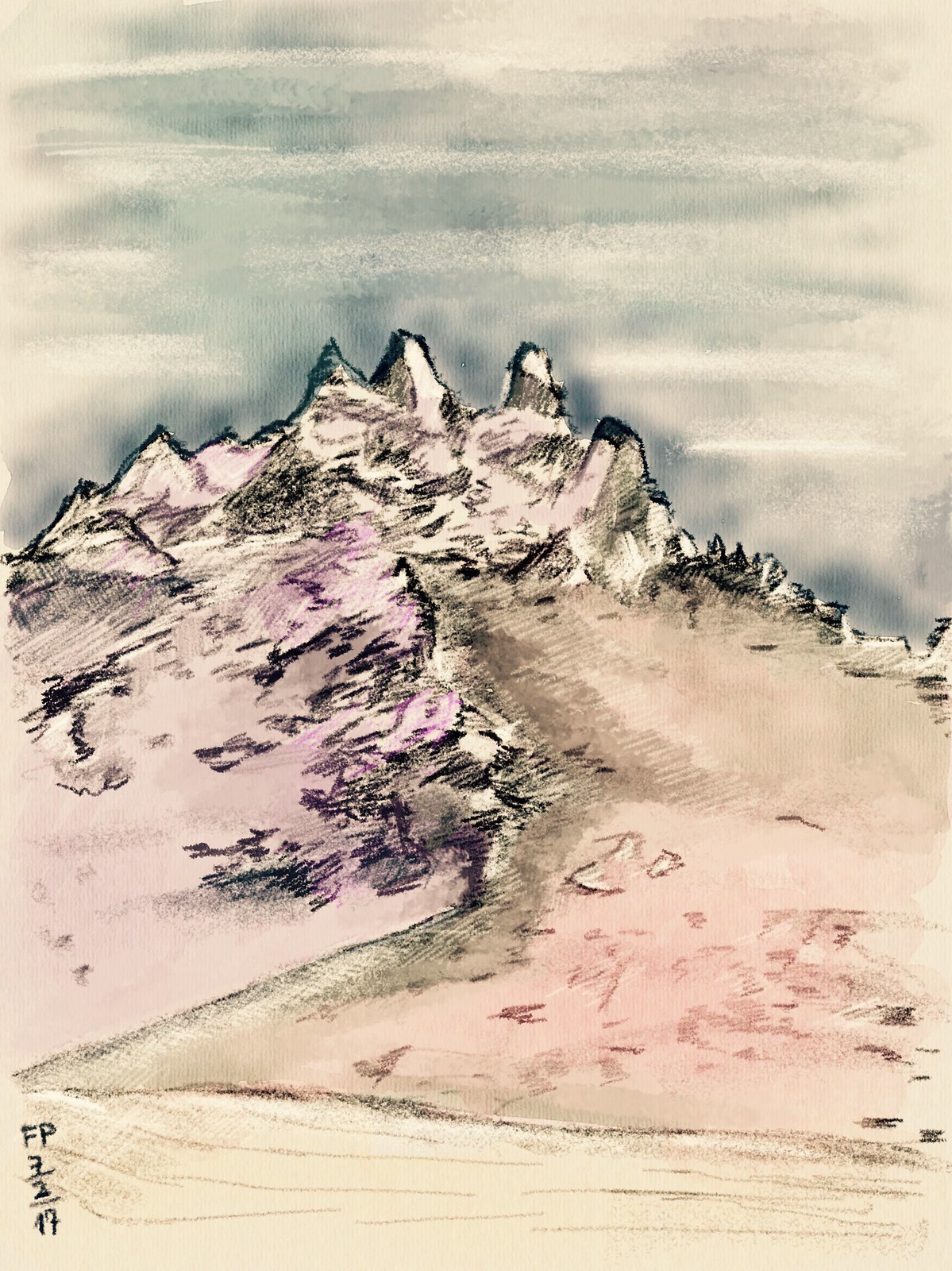This captivating painting illustrates an outdoor scene dominated by a majestic mountain. The artistic style is distinguished by its detailed and intricate composition, featuring bold black line work that accentuates the contours and shapes within the image. The mountain itself begins with a smooth, sand-like texture at its base, transitioning seamlessly into rugged, sharply defined peaks towards the summit. These peaks are particularly striking due to the pronounced black lines that outline them, creating a dynamic visual contrast. The sky above the mountain is rendered in muted tones of white and gray, adding an atmospheric quality to the overall composition. The image is devoid of any text, allowing the viewer to fully immerse themselves in the serene yet dramatic landscape.